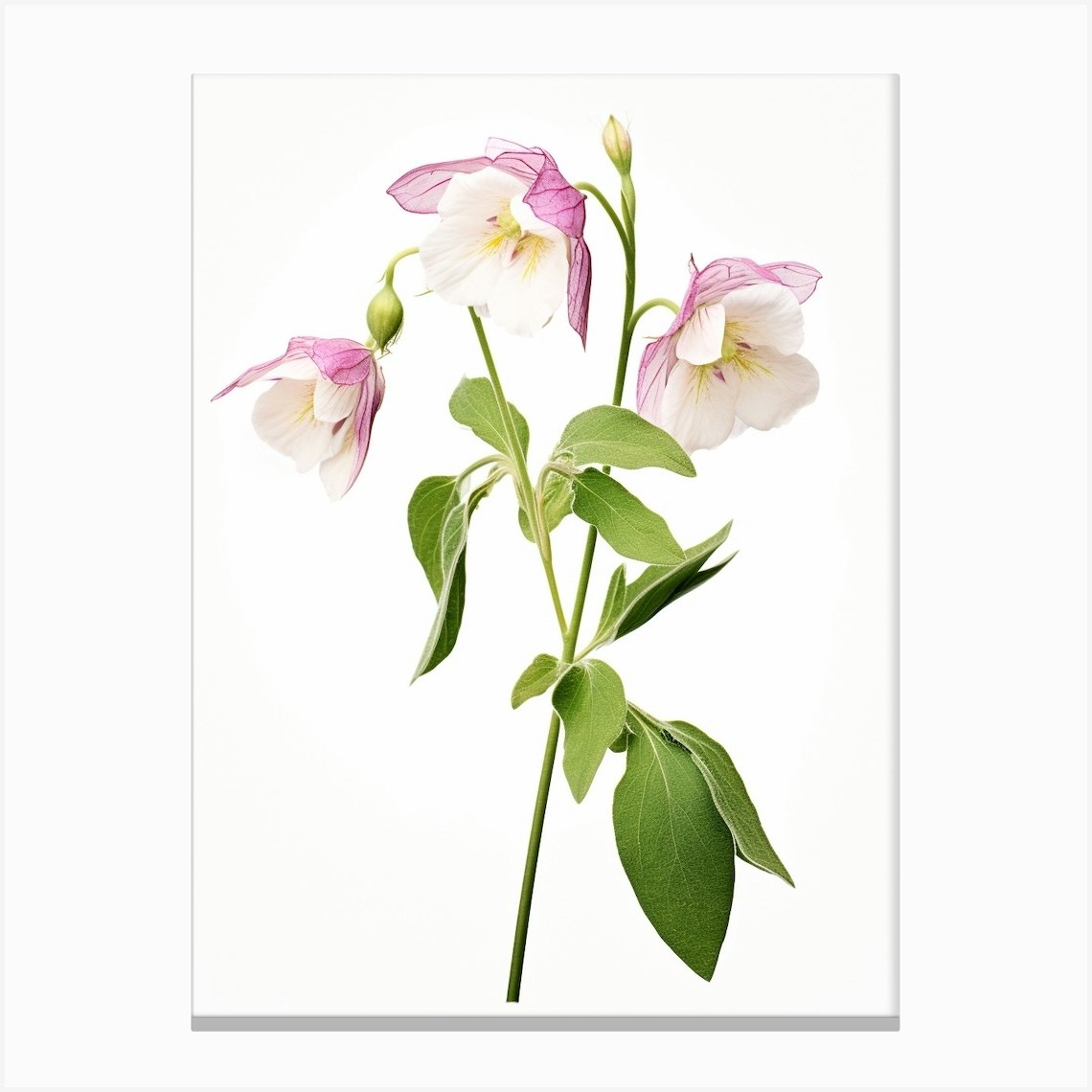This image showcases an artistic depiction of flowers against a vibrant white background, resembling a painted canvas. Central to the composition is a long green stem that extends vertically through the middle. This stem is adorned with multiple green leaves, with three leaves angling downward towards the lower right corner and more ascending leaves pointing upwards in the center. There is also a branch near the top left with four downward-slanting leaves.

Two prominent flowers emerge from the central stem, each positioned symmetrically on either side, facing downward. These flowers are characterized by their white petals and yellow centers, complemented by a large pink petal that cups each flower from behind. Additionally, there is a flower bud at the very top of this primary stem.

Off the side branch near the top left, a similar flower—white with a yellow center and encompassed by a pink petal—also droops downwards, accompanied by a nearby bud. The flowers, although depicted with vitality in their coloring, appear to be wilting due to their downward orientation. The entire floristry motif is set against a white expanse with a subtle gray sliver at the bottom, enhancing the visual starkness of the vibrant plant against its minimalist backdrop.